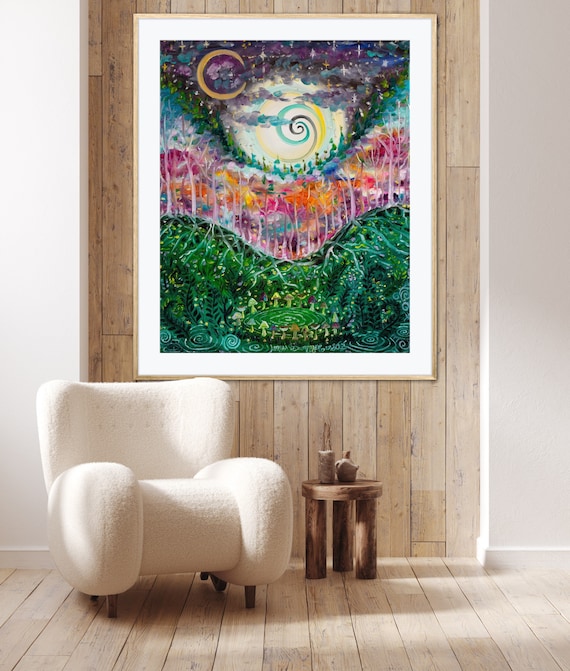The image depicts an indoor setting characterized by a grey wall with a very white trim at the bottom. Central to the scene is a section of the wall adorned with wooden paneling, acting as a focal point, upon which an abstract, multicolored painting is mounted. The painting features a whimsical landscape with green forest areas, white trees, vividly colored flowers, a crescent moon, spiraling skies in hues of blue, black, and yellow, and a starry backdrop. Below the artwork, the room’s light-colored wooden floor is visible.

To the right of the setup, there's a small, white fabric-upholstered sofa chair with four short wooden legs and a back peppered with ten dark holes. Accompanying this chair is a small wooden stool featuring three pegs as legs, serving as a side table. On this stool, there is a jug with a handle and a cork, as well as a small pot containing a plant with bare branches. Illuminating the scene is a light source coming from the upper left side. The overall décor, including the wooden elements and art, creates a cohesive and inviting interior space.